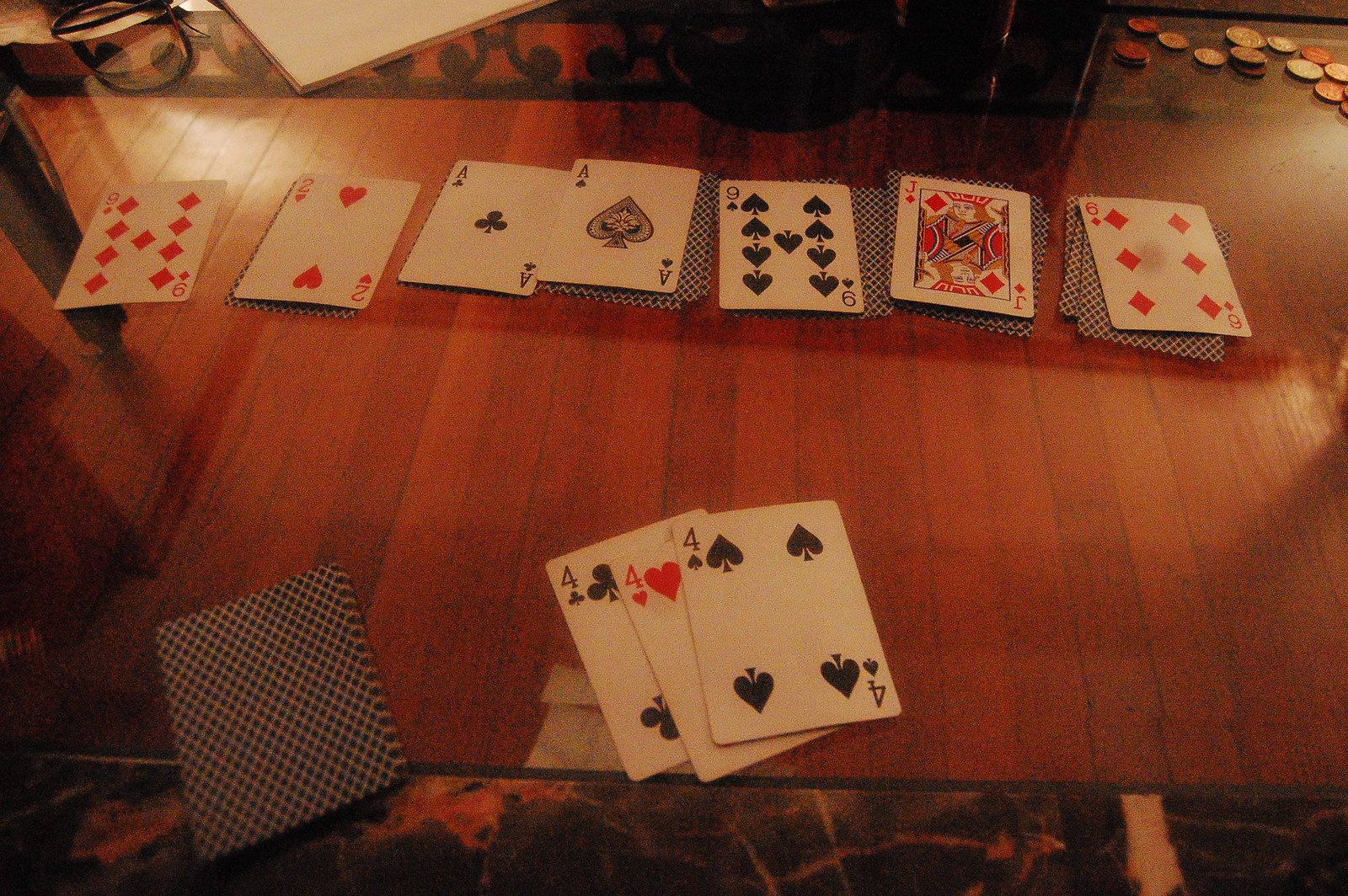A vibrant color photograph displays an intricate card game setup on a glass table, revealing the wooden floor beneath. On the upper half of the table, a neat row of playing cards lies face-up, showing a nine, a two, two aces, another nine, a queen, and an eight. Below these, several stacks of cards are positioned face-down, with one stack consisting of three fours visible. Scattered around the table are some copper pennies and silver coins, adding a touch of randomness to the orderly game setup. Light floods the scene from a nearby window, illuminating the arrangement. Notably, no players or hands are visible, leaving the focus solely on the cards and coins.